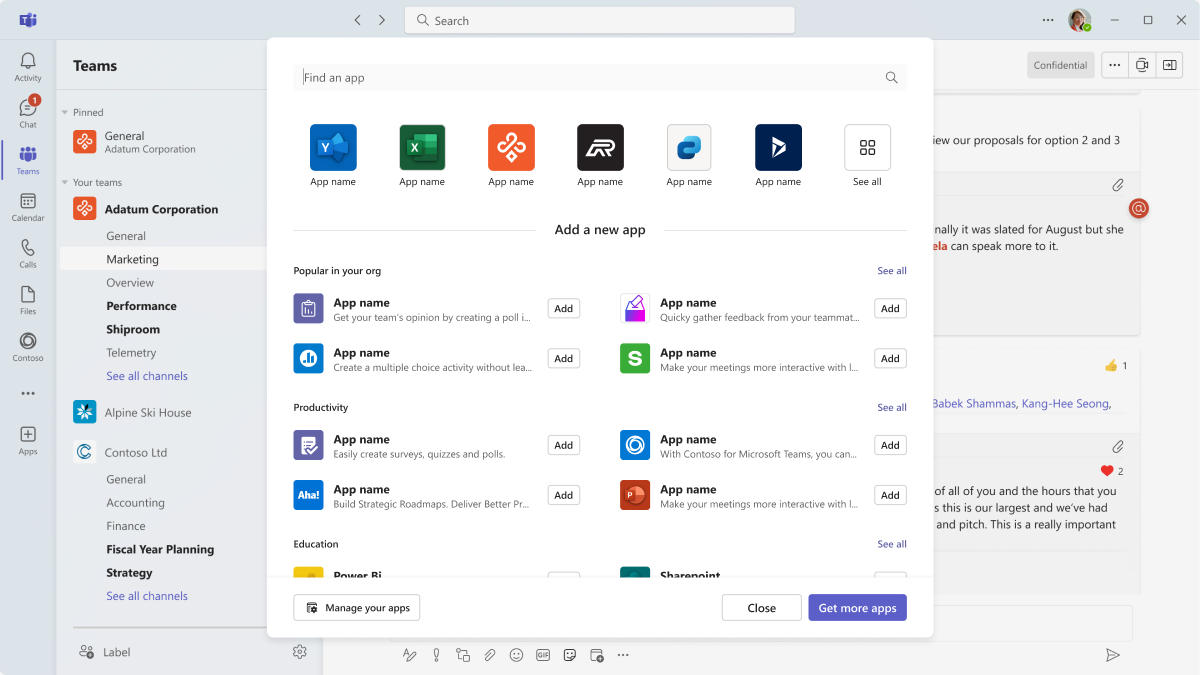This image showcases a pop-up window from a web-based productivity platform, likely part of a larger team collaboration system. The interface features a sleek design with a predominantly light gray color scheme.

On the top of the screen is a light gray search bar allowing users to quickly find specific content or functions. Along the left-hand side, there is a vertical dark gray navigation bar with several icons and categories identified, including 'Activity,' 'Chat,' 'Teams,' 'Calendar,' 'Calls,' and 'Contacts.' Each category is represented by a small illustrative icon for ease of recognition.

In the upper right corner of the interface, a user's profile picture is visible, indicating that the user is logged in. The central part of the pop-up window prominently displays a title, "Find an App," followed by a list of app names, which are available for selection. This functionality seems tailored for users who want to add specific apps to enhance their team's productivity. The apps are listed under different sections such as "Popular in Your Org" and "Productivity," featuring common workplace productivity tools. Another section titled "Education" offers a variety of educational apps.

Beneath this pop-up window, the underlying webpage, possibly related to a Q&A section, is slightly visible. Additionally, the main screen (behind the pop-up) shows navigation headers associated with specific teams or projects like "Price Your Teams" and "Alpine Ski House." Under these headers, multiple categories such as 'General Marketing,' 'Overview,' 'Performance,' 'Skip Room,' and 'Ship Room' are listed, suggesting a structured organization aimed at various team functions and projects.